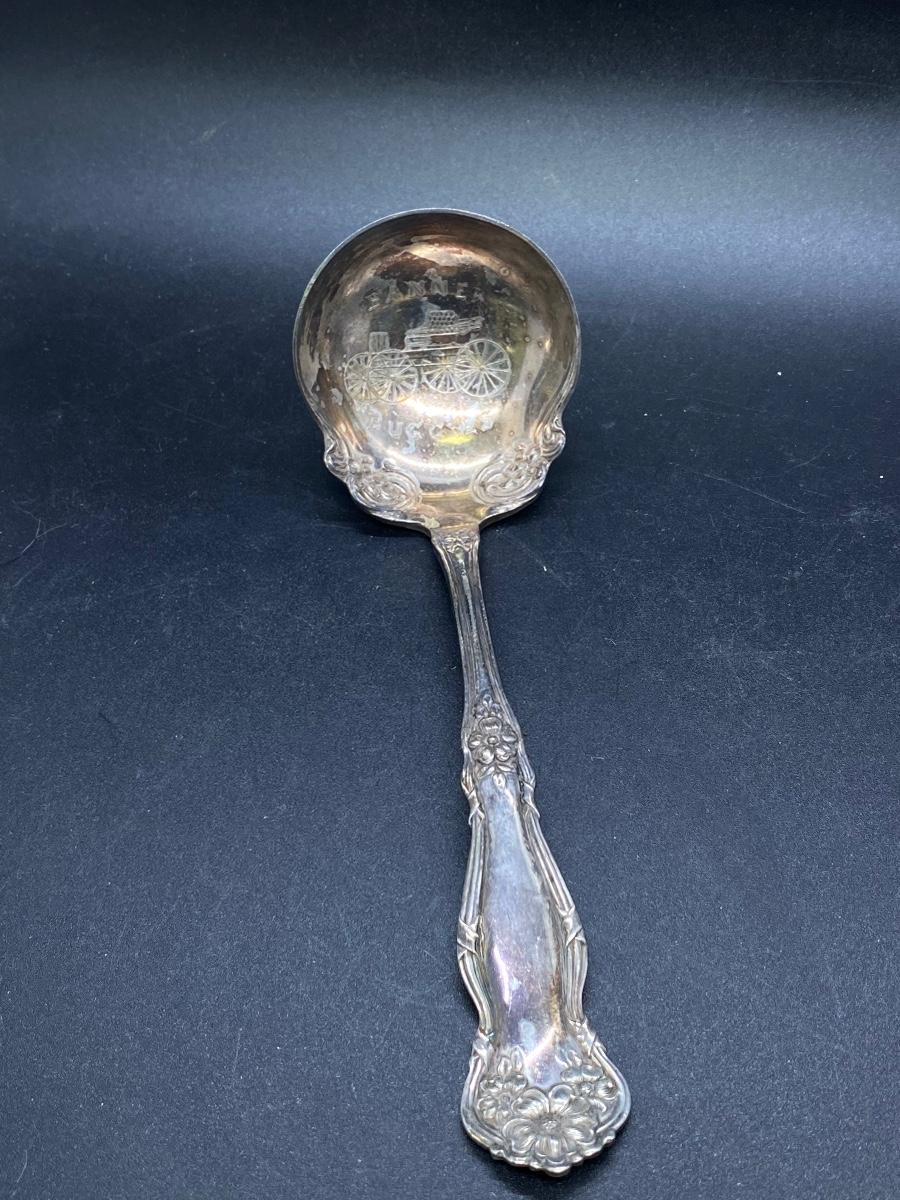This is a detailed photograph taken from above, showcasing a medium-sized antique silver spoon laid out on a blue background. The silver spoon is quite ornate, featuring intricate engravings along its handle, which include various flowers, notably roses with distinguishable petals. The spoon bowl is large and scallop-shaped, suggesting it could be used for serving punch, resembling a ladle more than a typical soup spoon. Inside the spoon bowl, there is an inscription depicting a steam engine or carriage, with some writing above, possibly reading "Banner." The spoon's surface shows signs of tarnish, further emphasizing its vintage and well-used nature. The design elements extend from the base of the handle to the top, making it a beautifully ornate piece likely intended to showcase its antique craftsmanship.